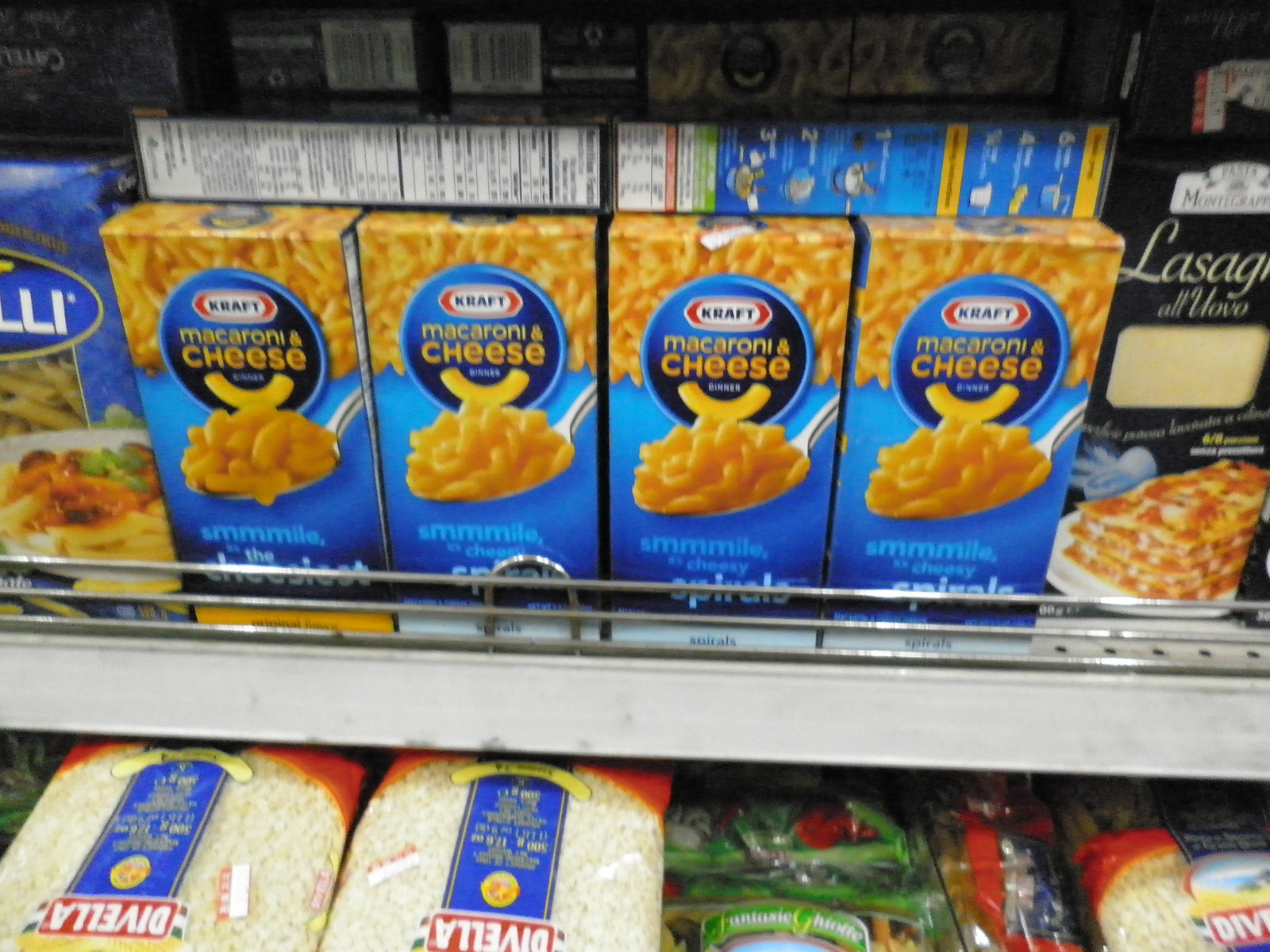The photograph captures a display of food items at a grocery store. Central to the image are four prominent boxes of Kraft Macaroni and Cheese arranged in the middle, with additional boxes stacked behind them. The iconic blue packaging features the standard brand logo and vibrant yellow images depicting the macaroni and cheese. To the right of the macaroni and cheese boxes, there are packages of lasagna sheets neatly positioned. Below the macaroni and cheese, several bags of what appears to be rice are visible, though the text is upside down and unclear. Additionally, there are cans or bags of green beans or a similar green vegetable situated in the lower section of the display.